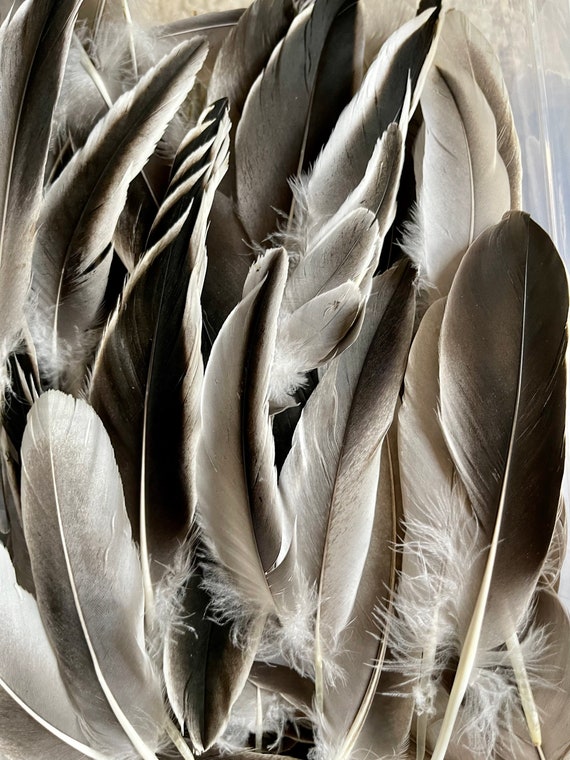The image depicts an intricate composition of numerous feathers, meticulously covering the entire frame. The feathers, varying in shades of dark grey, light grey, beige, and brown, overlap each other from multiple angles, creating a dense, textured pattern. Each feather is characterized by a distinct white central stem and delicate, white fringes along the edges. The overall effect is reminiscent of a detailed painting, capturing the feathers' subtle tones and intricate layering. With feathers of different sizes stacked atop one another, the image evokes a sense of natural elegance, much like the plumage of a pigeon.